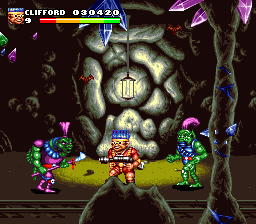The image appears to be a vibrant and colorful screenshot from a video or computer game with the title "Clifford 030420" displayed at the top. Set within a rocky cave environment adorned with both blue and purple crystals, the scene is illuminated by a hanging lamp. Three distinct characters are positioned under the lamp, which casts a dramatic light on them. 

The central figure features blue spiky hair, glasses, and a red uniform, holding a weapon. Flanked by two green-skinned characters, each donning different attire and sporting purple accents in their hair, they seem to be in action, possibly engaging in a tactical combat scenario. Despite the dark cave backdrop, the overall composition bursts with colors including fuchsia, green, blue, silver, brown, black, and yellow, creating a striking and visually engaging scene.